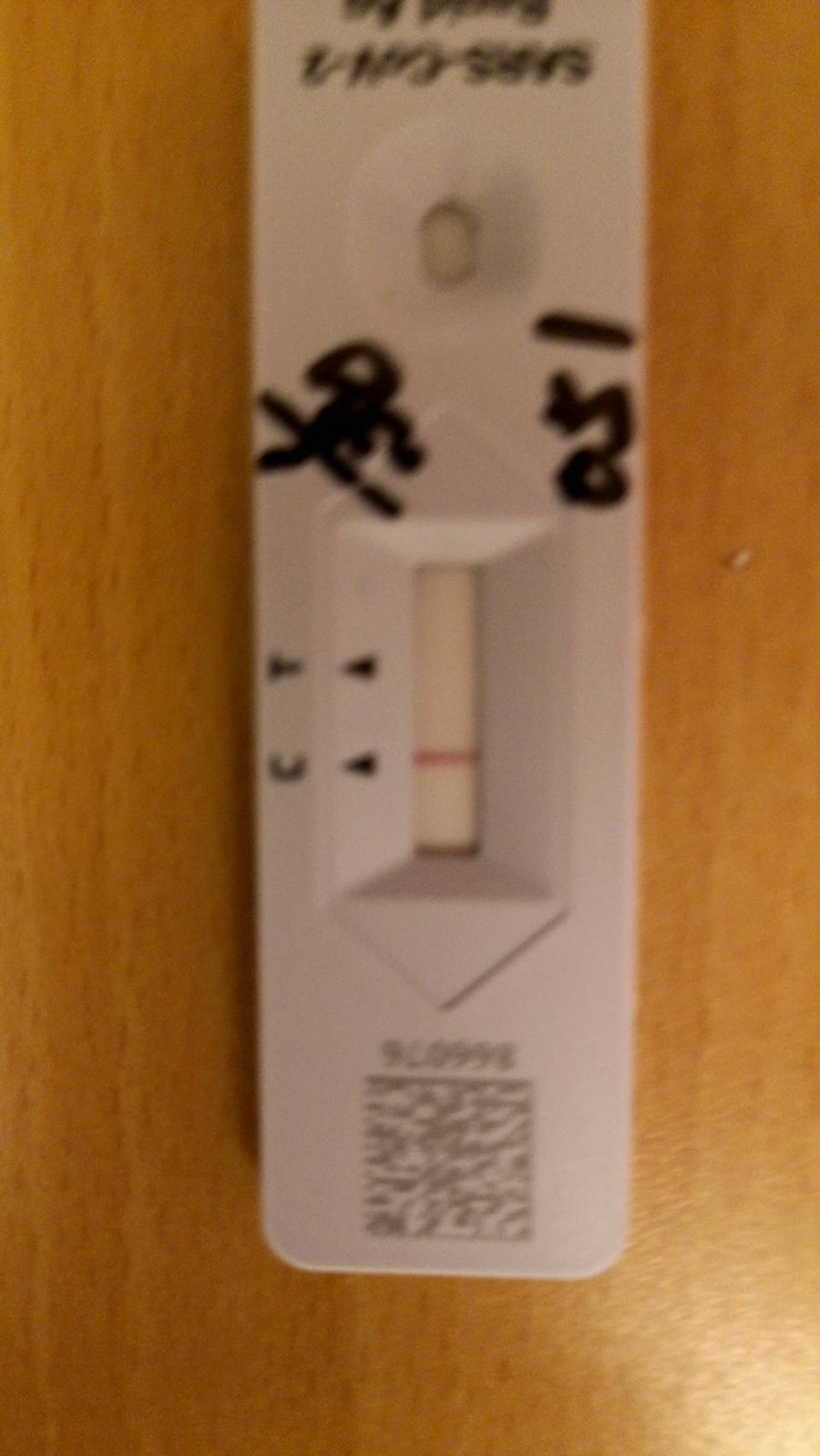An out-of-focus photograph captures a white plastic object resting on a wood grain surface. The object is marked with a handwritten note in black marker that reads "1/30" and "051." Upside down at the top, the text "SARS-CoV-2" is visible, followed by an unreadable section. There is a small, oval indentation on the surface of the object, possibly for inserting something. At the bottom of the object, an indicator with two black arrows points towards the letters "C" and "T." A red bar is positioned inside the indicator, aligned with the "C." Below this, there is a block of tiny, gray text that is unreadable along with the number "866-076" also in gray. The image's lack of focus obscures finer details.